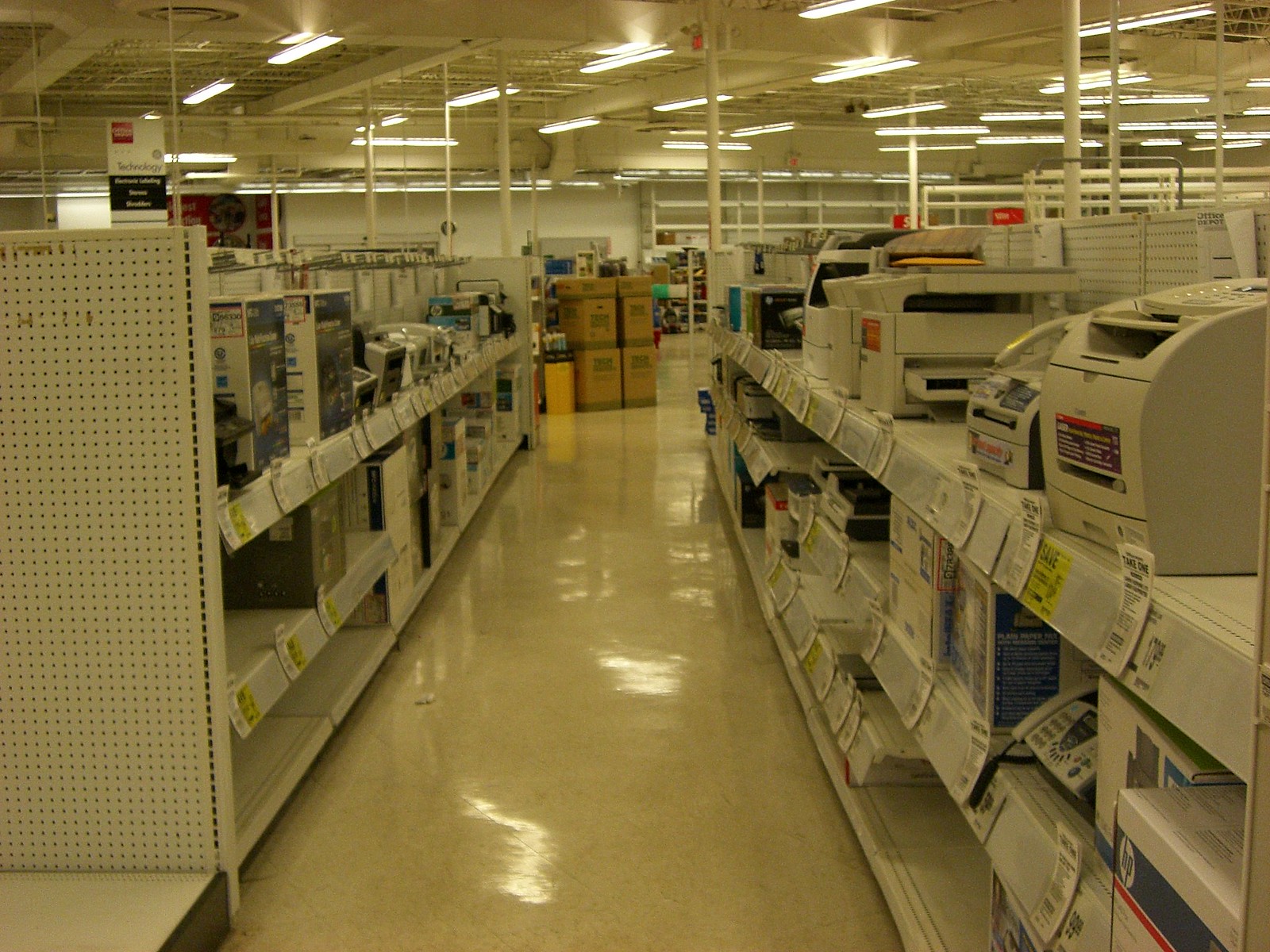The image depicts the interior of a computer or technology store with a modern, industrial design. The store features an off-white, shiny stone floor and an exposed metal ceiling with visible ductwork and hanging halogen lights, giving it an open and contemporary feel. Directly in front of the viewpoint are white wire shelves, organized into three levels. On the top shelf sits a beige printer, accompanied by small sections containing product information and pricing details. Rows of shelves filled with various computer equipment and technology products are visible throughout the room. In addition, boxes of paper are stacked on some of the shelves, catering to customers looking for bulk paper supplies. The overall scene presents a well-stocked, organized store dedicated to a wide range of computer and technological needs.